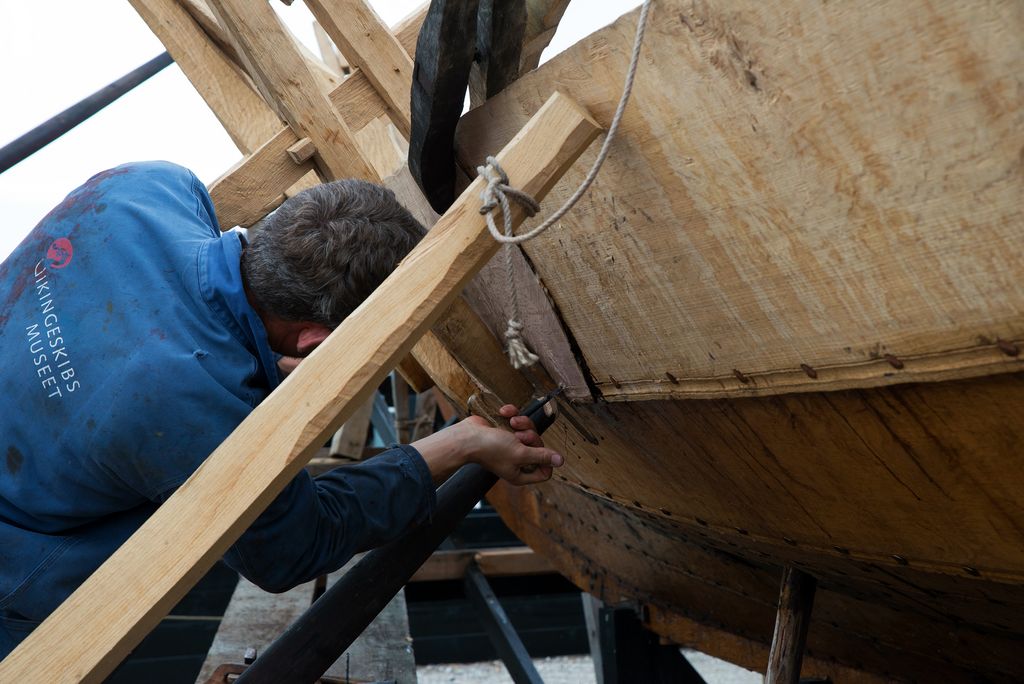This detailed color photograph captures a man, whose face is not visible, diligently working on a large wooden structure that appears to be a boat, possibly displayed at a museum. The man is facing right, deeply focused on his task, with short grayish-brown hair visible from the side. He is wearing a blue coverall uniform that reads "VIKINGESKIBS MUSEET" in white letters on the back, accompanied by a red circular logo, indicating his affiliation with a museum dedicated to Viking ships. The wooden boat is elevated and supported by wooden poles, ensuring it's kept off the ground. The man is holding a tool, possibly used for boring holes, suggesting he might be adding some type of liquid to the boat's structure. Adjacent to the boat is a long piece of wood tied up with rope, leaning against the boat and tilting upwards to the right. This detailed scene highlights the meticulous care taken in preserving historical artifacts.